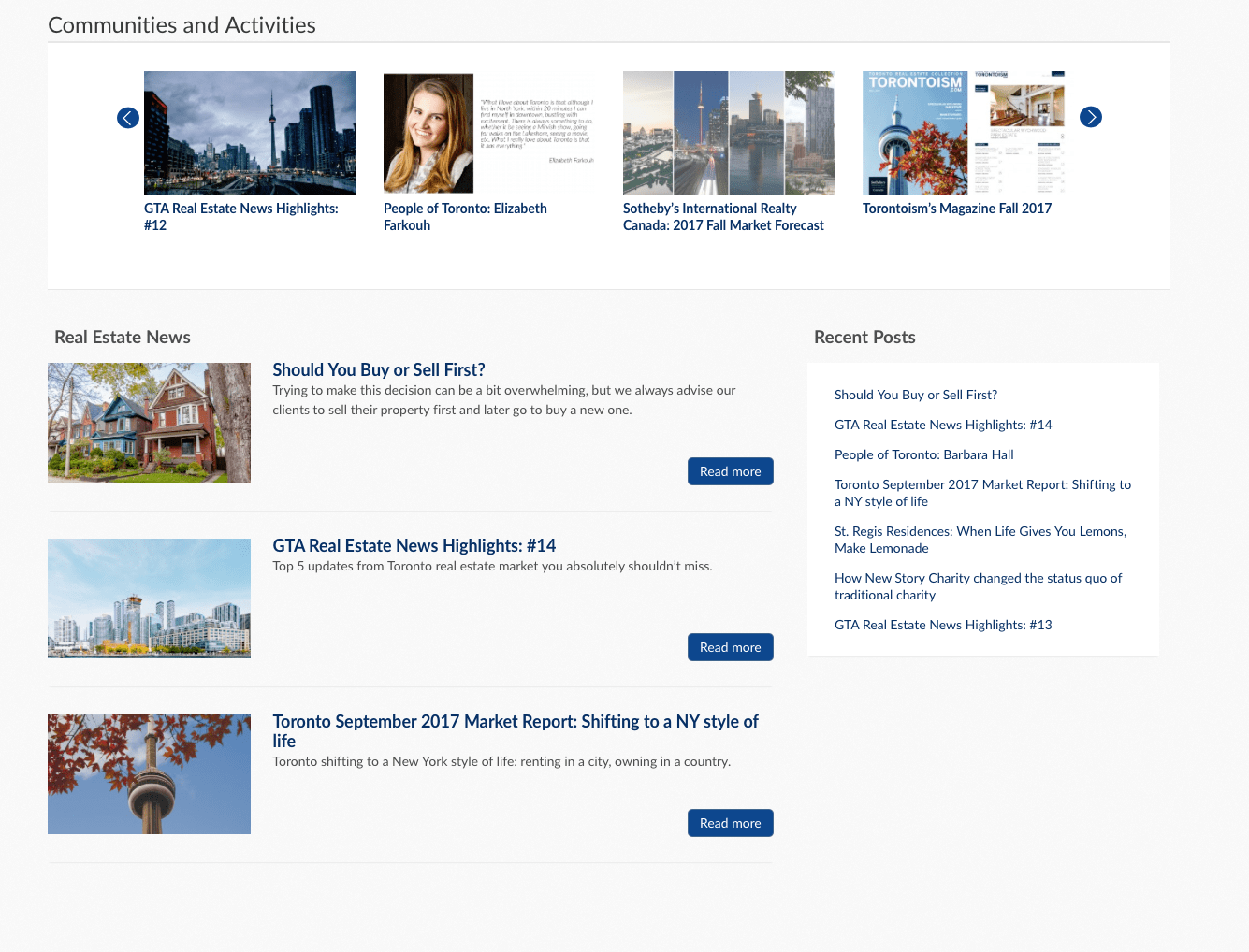This is a cropped image of a web page displayed in desktop mode, featuring a very light gray primary background color. Accenting the layout, the upper banner and the recent posts list on the right are set against white backgrounds.

The top banner, labeled "Communities and Activities," showcases a horizontal row of four pictures: a cityscape, a portrait of a woman, a collage of four vertical city shots, and a magazine cover titled "Torontoism" with accompanying text that is illegible at this resolution. Each image has blue hyperlinks below it, leading to corresponding articles. On either side of this banner, there are left and right navigation arrows with white icons, allowing horizontal scrolling through additional articles.

The main section of the web page is dedicated to real estate news. It includes three articles, each with a clickable "Read More" button in blue located at the bottom right of the entry. The first article is titled "Should You Buy or Sell First," the second is "GTA Real Estate News Highlights Number 14," and the third is "Toronto September 2017 Market Report: Shifting to an NY Style of Life." Each title is accompanied by a brief one- or two-sentence blurb providing further elaboration on the content.

To the right of this main section is a "Recent Posts" list, featuring seven additional articles that are not highlighted in the main section, all of which are clickable for more detailed reading.